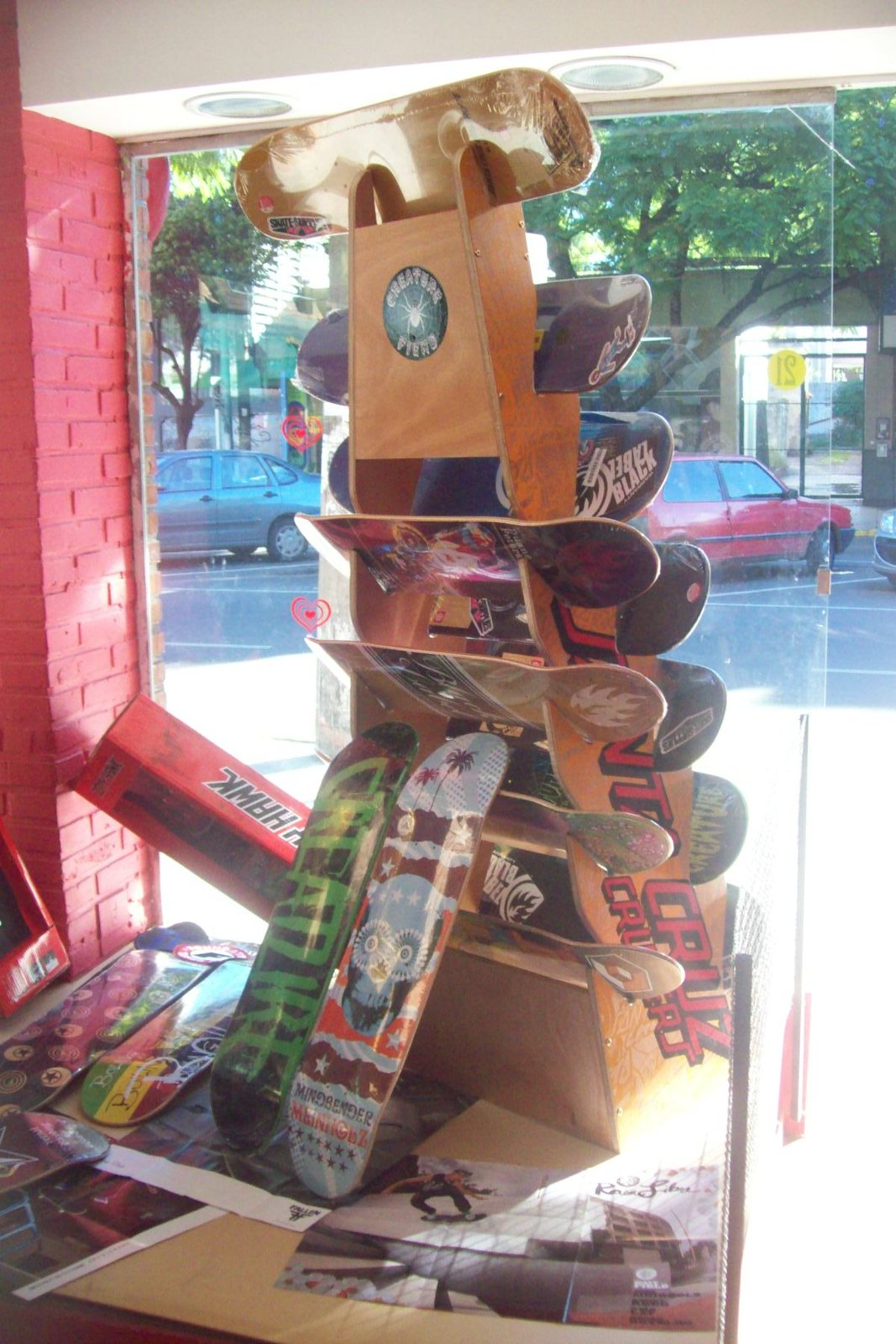This vibrant photograph captures the interior of a skateboard shop as seen through its front display window. Dominating the view is a large, light brown wooden rack shaped like a pyramid, designed to hold numerous skateboards. Slotted into the rack at various angles are a total of twelve skateboards: seven on the front in ascending rows, five on the back, and an additional skateboard perched at the very top. Each skateboard boasts distinct colors and patterns, with one notably displaying the word "Santa Cruz." To the left, a red brick wall painted in a bright hue frames the scene, with a red box marked "HAWK" in black letters leaning against it. Beyond the glass, angled parking spots are visible, occupied by a red and a silver car, and the area is shaded by trees, enhancing the cozy, bustling atmosphere of the shop.